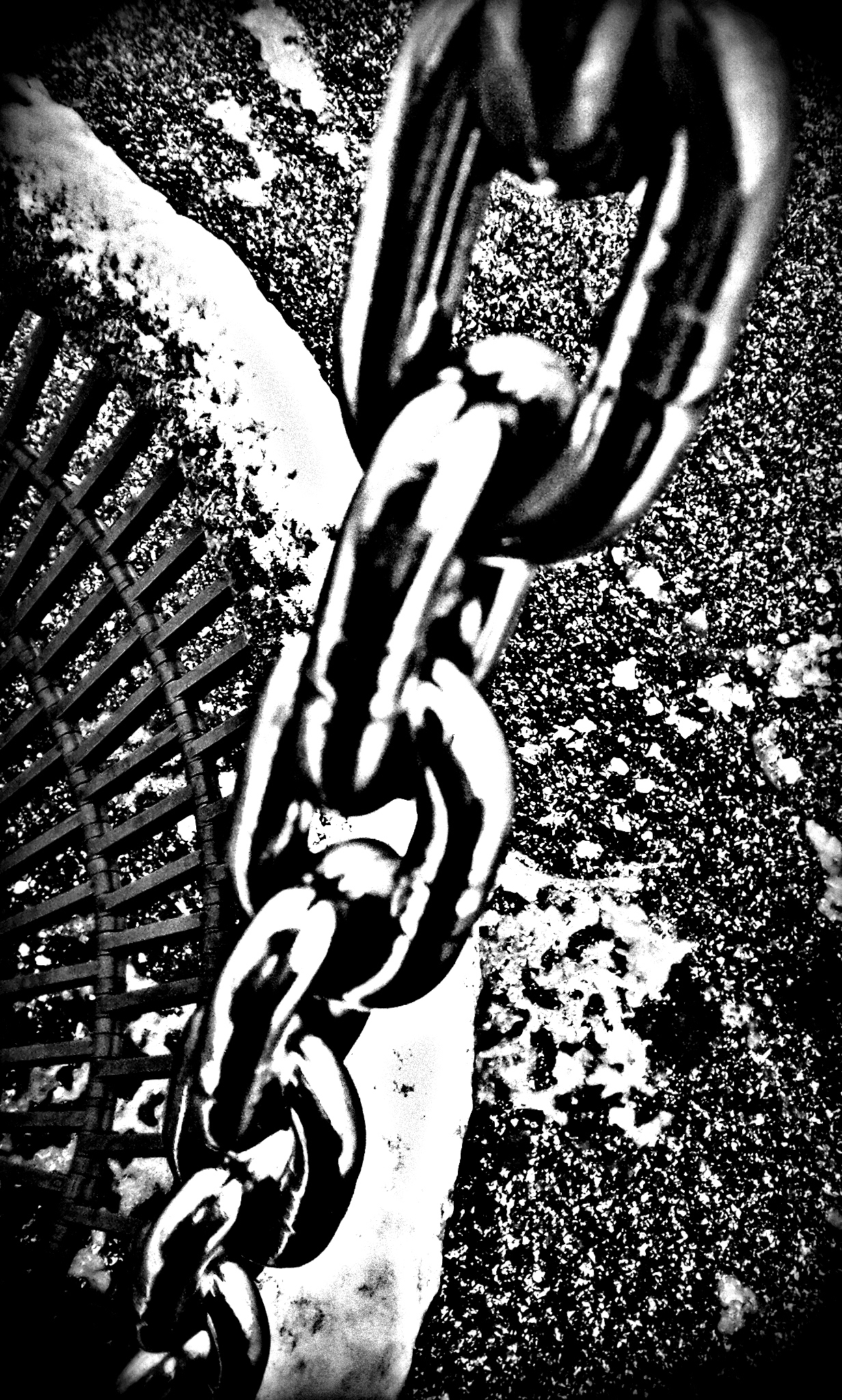This black and white photograph, rendered with a heavy filter, captures a surrealistic close-up of a metal chain with significantly large, shiny silver hooks. The chain stretches diagonally across the vertical image from the upper right corner to the lower left. Dominating the foreground, the chain partially obscures the background, which features a circular, black metal object on the ground. This circular shape, possibly a storm grate or an architectural element, is covered in white snow-like powder and flanked by spokes made of black wrought iron. The ground beneath and around this object is speckled with a white, crusted substance, suggesting either snow or a weathered stone texture. To the right, the scene transitions into a gravel or stone surface, adding to the textured ambiance of the image. The overall composition and the heavy use of black-and-white filtering lend the photograph a unique, almost artistic feel, making it difficult to discern the exact nature of some elements.